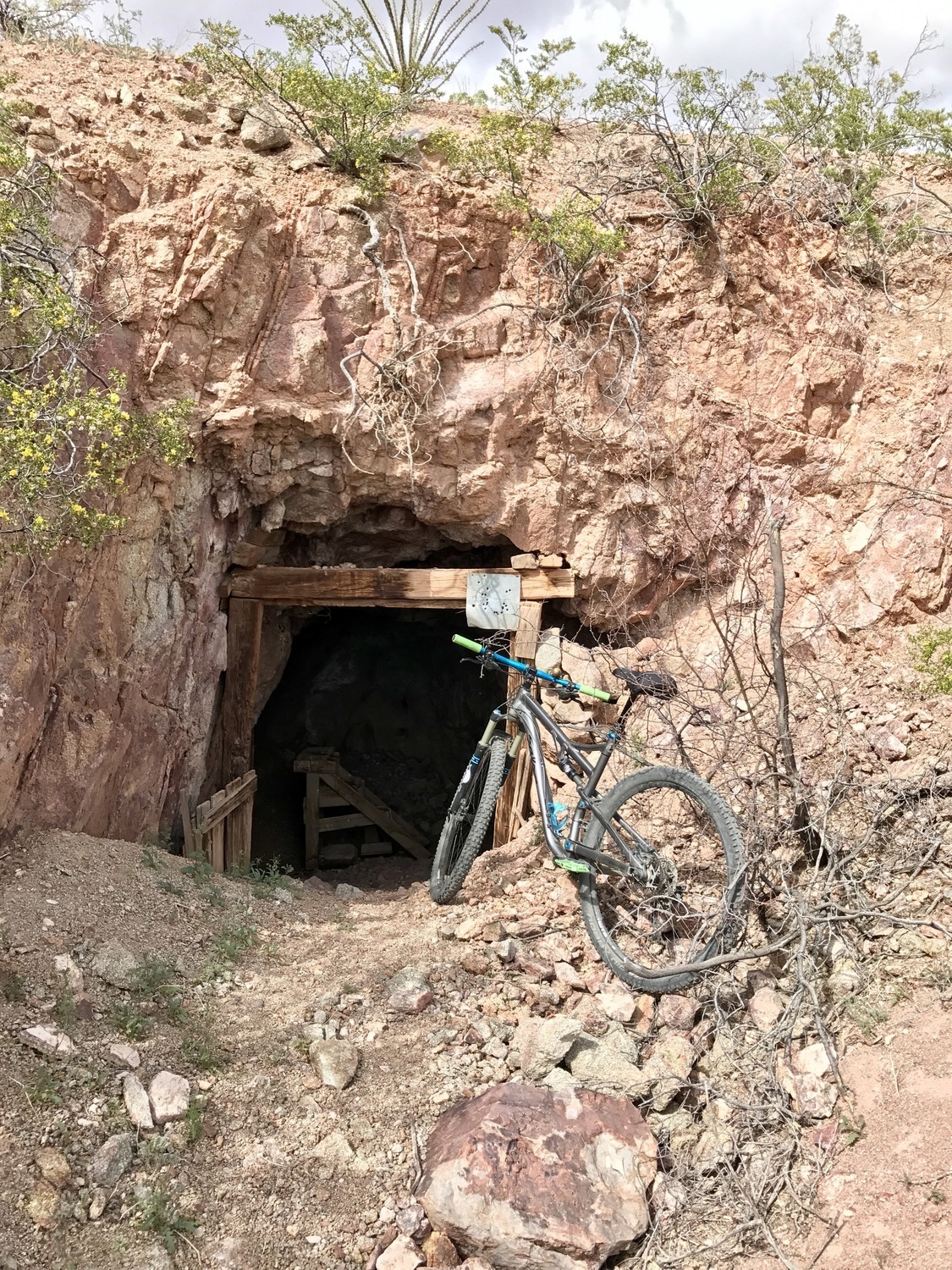This photograph captures the rugged entryway to a cave-like structure nestled into a rocky cliffside. The terrain is harsh and barren, dominated by rock, dirt, and clay, with sparse vegetation including some plants with exposed roots and a solitary plant with yellow flowers on the left. The cave's entrance is reinforced with wooden supports, resembling an old mine shaft or perhaps a makeshift doorway. This opening reveals a dark interior, with just enough visibility to hint at features like a potential staircase or railing inside. In front of the gate, a blue, green, and black mountain bike is parked, emphasizing the rough and adventurous nature of the location. The scene vividly depicts an isolated and mysterious cliffside passageway, devoid of any human presence beyond the parked bicycle.